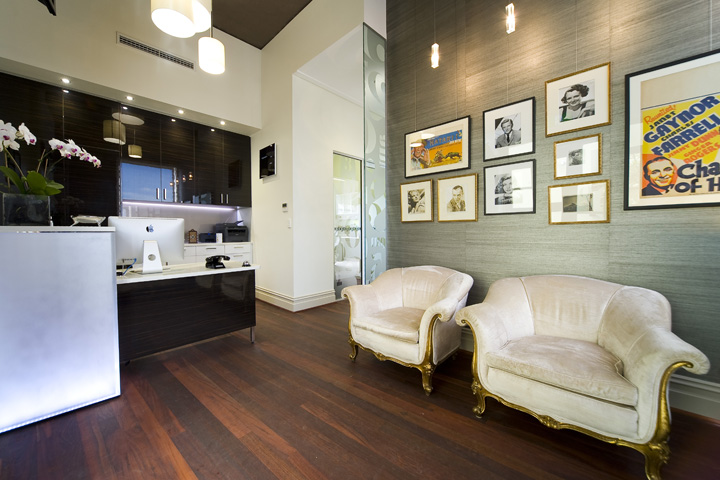The image depicts a stylish and welcoming reception area, most likely part of a dental clinic. The setting exudes a modern and inviting atmosphere with its open layout and tasteful interior design. The right-hand wall is painted in a soothing green hue and adorned with numerous photographs and artwork, including movie posters and images of vintage movie stars, giving the space an artistic flair. Below the artwork, there is an off-white loveseat with gold accents, accompanied by a matching chair.

The room features elegant wood flooring and strategically placed hanging lamps that contribute to the well-lit, cozy environment. A sleek black desk with a white top, which holds a silver Apple iMac computer, is situated against a black wall on the far side. Adjacent to the desk is a white counter displaying a vase with flowers, adding a touch of freshness.

On the right-hand side, in the corner, there is a door that leads to another room, through which one can glimpse equipment indicative of a dental office. This confirms that the aesthetically pleasing space is indeed the reception area of a dental clinic.